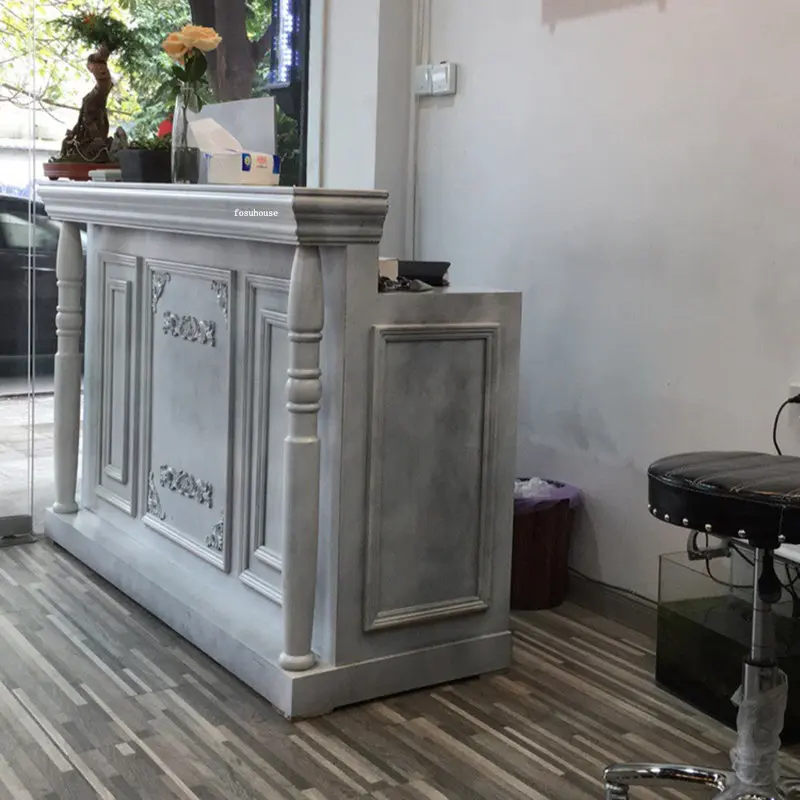The image depicts the interior of an establishment, likely a hairdresser’s salon, featuring a prominent front desk made of light gray material with intricate wood ornamentation and molding. This counter, reminiscent of a bar with a fold-back extension supported by two pillars, has rectangles carved into its center and sides, with a floral pattern adorning the middle section. Near the front desk, stands a big glass window that offers a view of the outdoors, revealing a piece of a car door and a leafy tree. 

On top of the desk, there's a neatly arranged display including a vase holding a rose, a box of tissues, a small plant resembling a bonsai tree, and decorative flowers. Behind this desk, one can also spot a metallic trash can and a terrarium or aquarium-like box with a gray base and clear top section. Adjacent to the desk, there is a black rolling chair with a cushioned seat and an adjustable frame, supported by a silver stem and five metal feet with wheels. The room's wooden floor showcases a blend of light and dark brown slats, adding a warm touch to the modern, clean aesthetic of the space. Other notable items in the room include a thermometer on the wall behind the desk, and off to the right side, nearly out of the picture, is another stool with similar design features.